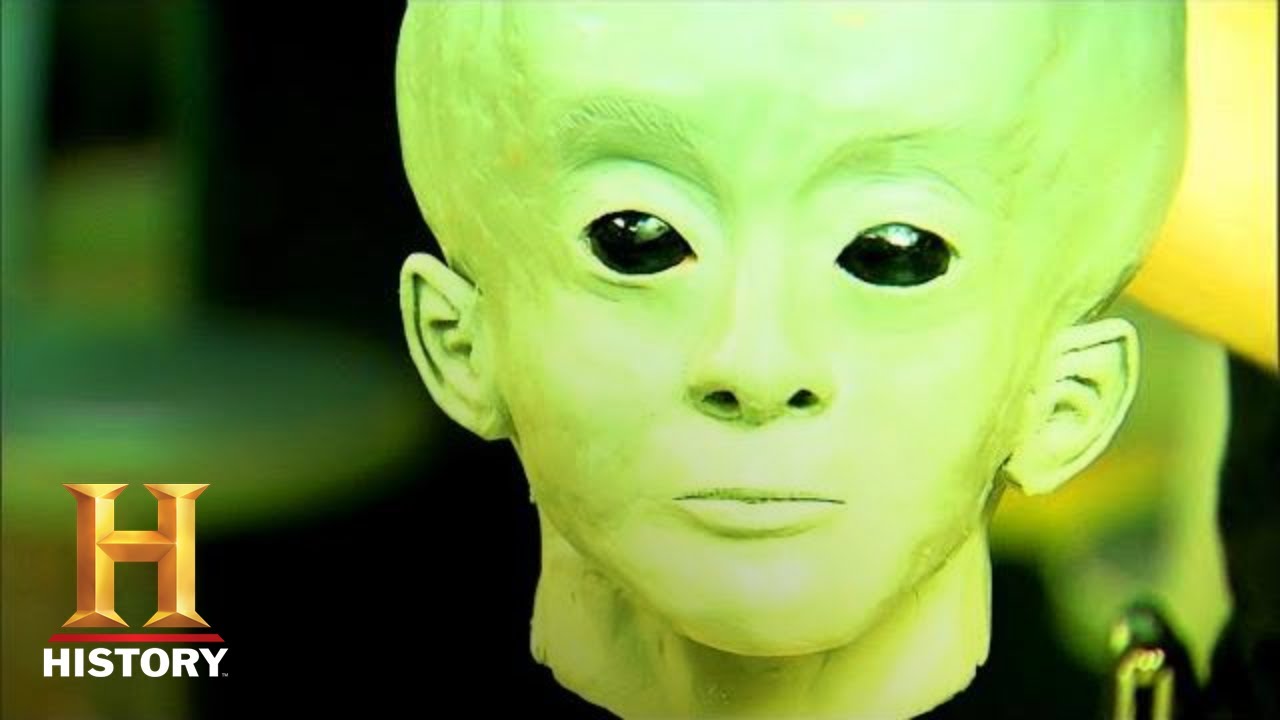This image features a computer-generated rendering of an alien with a distinct appearance. The focal point is a large, bald green head with a very pronounced, rounded shape. The face is hairless with pointed ears and a chin that tapers to a small point. The alien’s eyes are black and beady, devoid of eyelashes or creases, and its mouth is closed.

In the bottom left corner of the image, there is a gold letter "H" underlined in red and accompanied by the word "HISTORY" in white capital letters, indicating a possible association with the History Channel. The background of the image is blurred, featuring a mix of green, black, and yellow colors, which predominantly surround the alien figure. The contrast of these blurred background colors helps to emphasize the alien's distinct features.